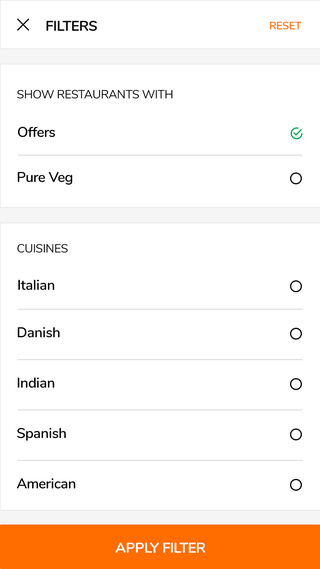The screenshot displays a mobile phone interface for a restaurant-filtering feature. At the top left, there is an 'X' icon for closing the filter menu, and a section for various filters. On the top right, "Reset" is written in orange letters, allowing users to reset their filter choices. Below is an option labeled "Show restaurants with offers," indicated by a green circle with a checkmark.

The section titled "Cuisines" lists several cuisine options including "Pure Vegan" (unchecked), "Italian" (unchecked), "Danish" (unchecked), "Indian" (unchecked), "Spanish" (unchecked), and "American" (unchecked). At the bottom of the interface, a prominent orange button says "Apply Filter." 

The current state shows that while the user is interested in restaurants offering promotions, they haven't selected any specific cuisines, suggesting flexibility in their food preferences. The interface appears straightforward and user-friendly, enabling easy navigation and selection.